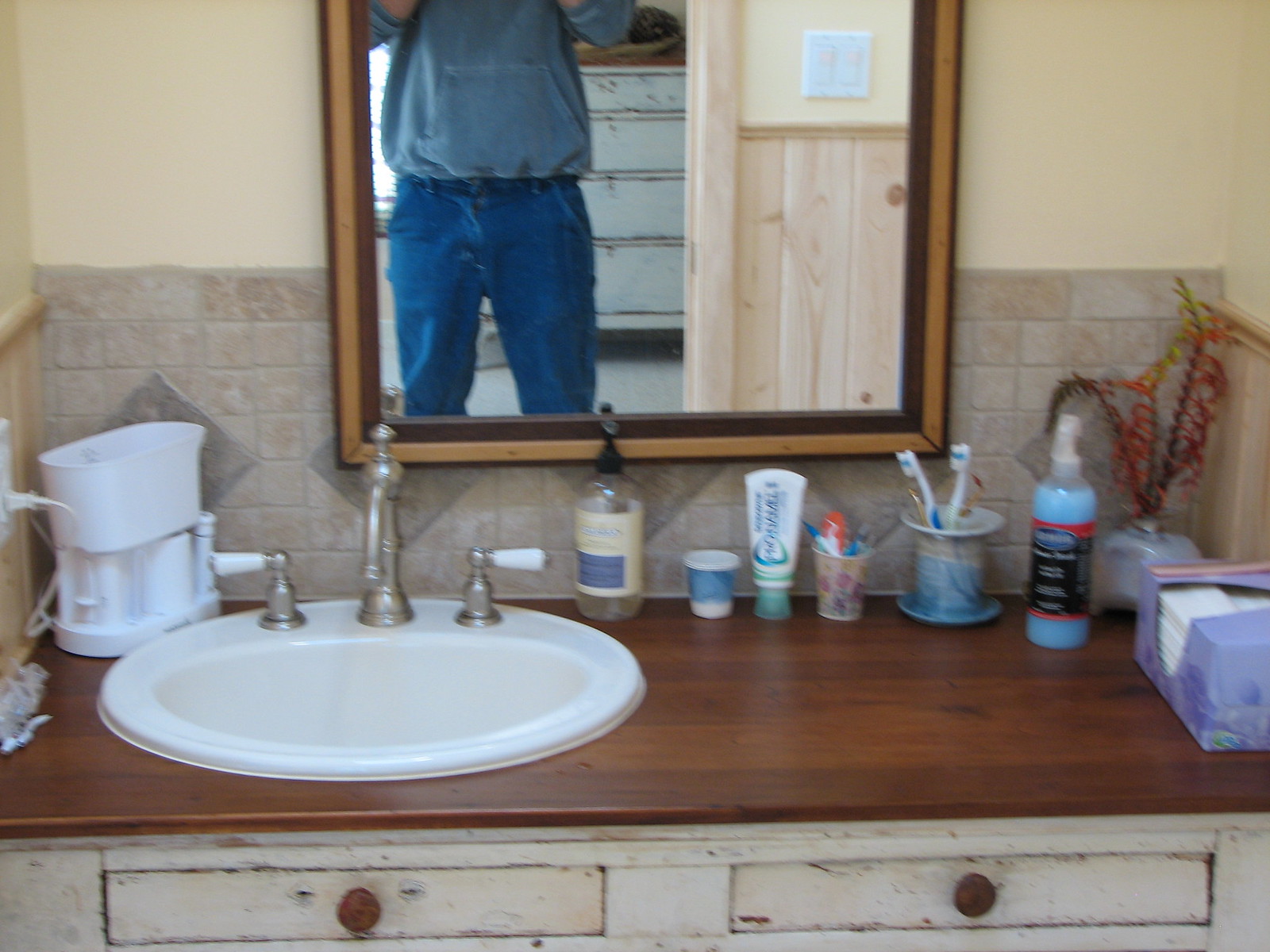A male, identifiable by his body shape and clothing, is taking a selfie in a bathroom mirror. His face is not visible, but he is dressed in blue jeans and a light blue long-sleeve shirt, with his elbows bent as he holds a camera or phone. The bulk of the image features an antique white sink and cabinet structure. The front of the cabinet has two slim rectangular drawers with dark brown handles, and the countertop is a dark wood grain with light knots, adding a rustic touch. 

A round sink sits to the left, with silver or aluminum fixtures and white, possibly ceramic, handles that extend outwards. Above the sink hangs a square mirror with a light brown border, reflecting a dresser and a cream-colored wall in the background. The wall itself is cream-colored, with decorative square and rectangular tiles covering the bottom third and extending behind the mirror. 

The countertop is cluttered with toiletry items such as soap, toothpaste, toothbrushes, and lotion, featuring various shades of yellow, white, and blue. In the back right corner, a decorative plant sits in a round holder, with a box of Kleenex placed above it. To the far left, plugged into a wall socket, is a white tooth-cleaning device, possibly a Waterpik. The overall setting suggests a cozy and personalized bathroom space.